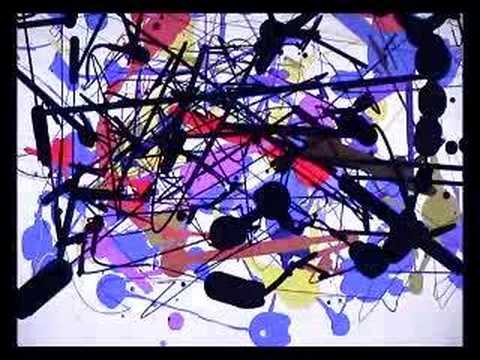The image features a rectangular abstract painting on a white canvas, bordered by a thick black frame. The predominantly white background is speckled with light gray and covered with a myriad of colorful streaks and dots, creating a chaotic yet intriguing visual texture. Black lines crisscross the canvas, forming a dynamic web, occasionally curving into more fluid shapes. Amidst the black lines, hues of purple, blue, red, and some yellowish-green and brown are dispersed throughout. Notably, there are elements that slightly resemble objects: a jellyfish-like shape with a string in the bottom left corner and a blue object with a red top in the top right corner. The painting seems to lack a central focal point, instead immersing viewers in an explosion of color and form, suggesting perhaps a childlike spontaneity. The abstract design and vibrant color palette dominate the scene, with layers of purple and blue receding into the background, covered by more prominent reds and blacks.